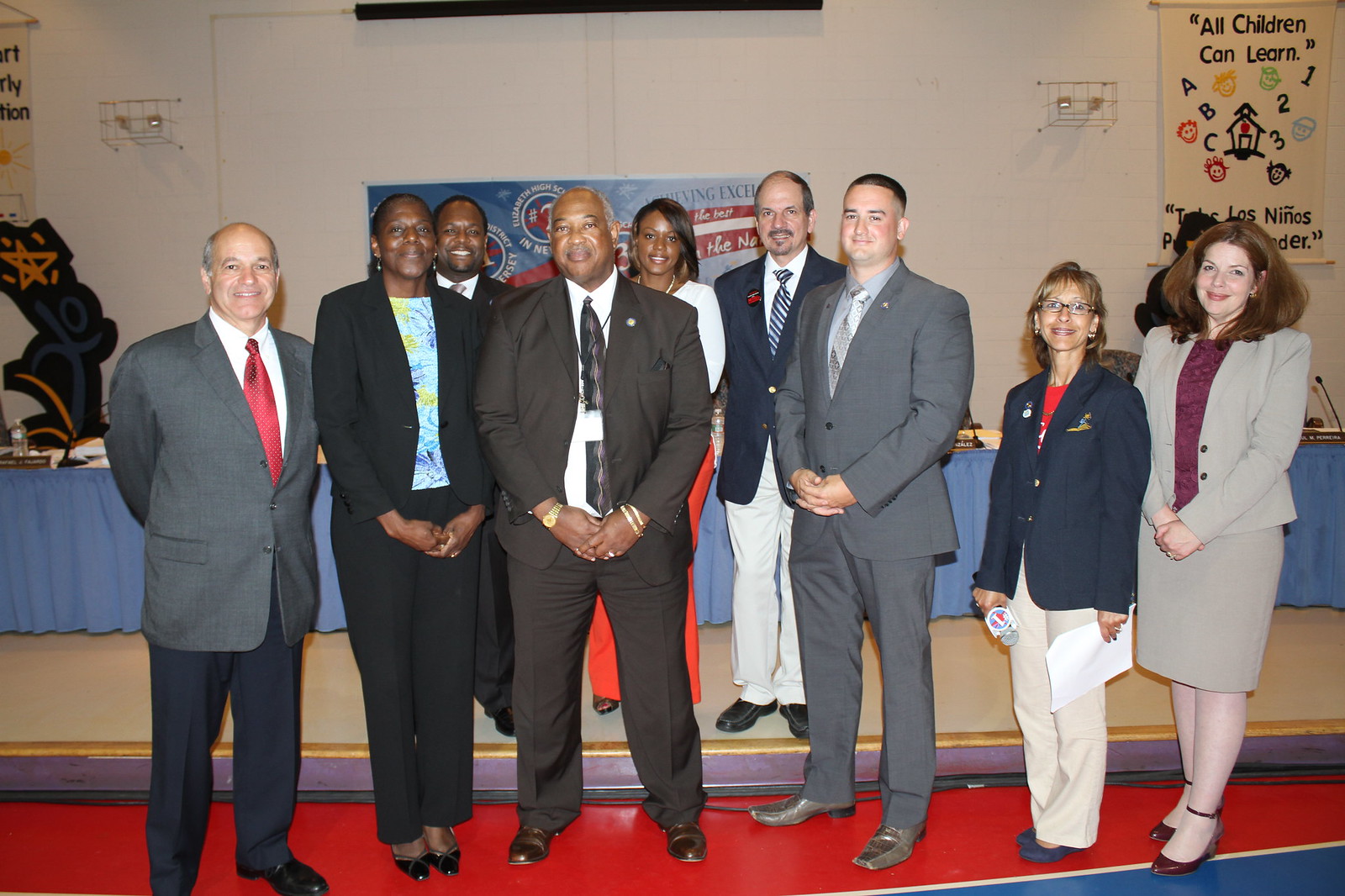In this indoor image, a diverse group of men and women are standing centrally on a multicolored gymnasium floor, appearing to pose for the camera. All individuals, dressed in business attire, including suits, sports coats, slacks, dresses, and high heels, stand in front of a backdrop featuring blue tables draped with tablecloths and various posters, one prominently displaying the slogan "All Children Can Learn." The background, which resembles an educational setting, also includes decorative elements like an orange star and cartoonish images of children, ABCs, and 123s. Among the group, one woman is seen holding a microphone, and several individuals are smiling directly at the camera, creating a unified and welcoming atmosphere.